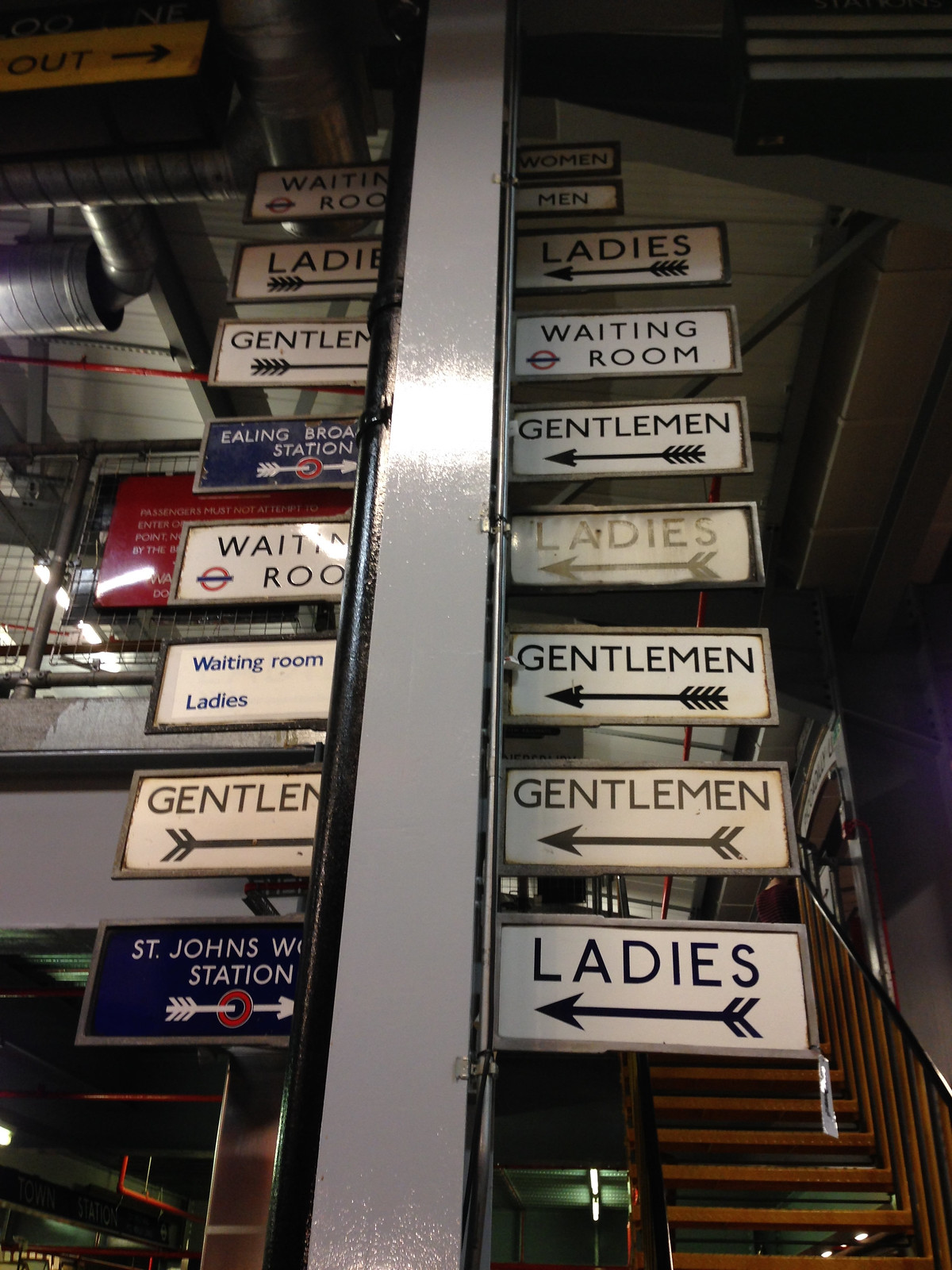The photograph depicts a close-up of a vertical I-beam, painted gray with black trim on either side, originating from the floor. Attached to the beam are numerous signs with directional arrows pointing both left and right, displaying somewhat confusing directions. Some of the text includes "Waiting Room," "Ladies," "Gentlemen," and partially cut-off names like "Ealing" and "St. John's." The signs guide to various locations such as waiting rooms and restroom facilities for men and women. In the background, there are brown steps leading upward, and large industrial piping runs along the ceiling. A chain barrier, indicating an off-limits area, is also visible. The setting appears to be an indoor, possibly a train or subway station, with a window visible at the top and an orange sign that says "OUT."